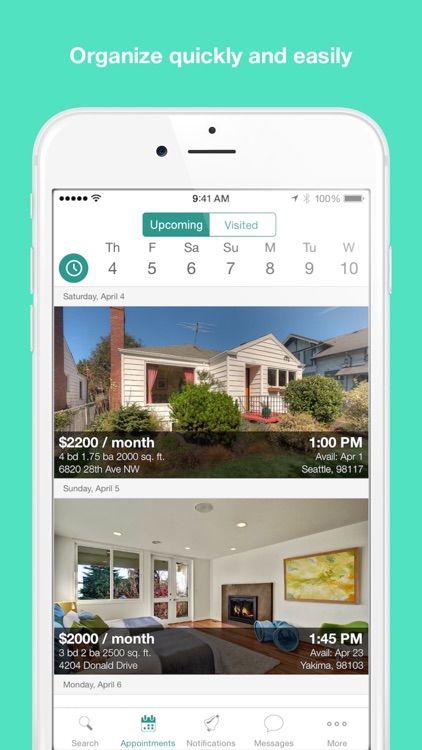Screenshot of a Bright Green Page Featuring Rental Properties on a Mobile App

This image displays a screenshot of a mobile application interface with a vivid green background. At the top, a prominent white header reads "Organize quickly and easily." Visually centered is a white phone graphic that shows an app screen. The app itself is organized with two tabs at the top: a green tab labeled "Upcoming" and a white tab labeled "Visited" positioned to its right.

Beneath these tabs is a horizontal row that abbreviates the days of the week, starting from Thursday through to Wednesday. The app screen currently highlights two rental property listings. The first property, with a $2,200 monthly rent, showcases a detailed description and a thumbnail image of a tastefully furnished living room. This property is noted to have 4 bedrooms and 1.75 bathrooms with a total living area of 2,000 square feet, and has a viewing time scheduled at 1 PM.

Overall, the app interface is designed to be visually engaging and user-friendly, facilitating easy organization of rental property information.